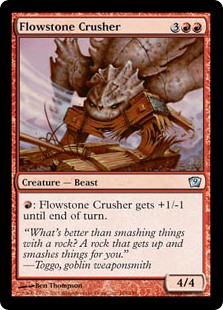The image depicts a rectangular Magic: The Gathering trading card named Flowstone Crusher. The card features a distinctive brown color with a black outline and measures taller than it is wide. At the top of the card is the name "Flowstone Crusher," while the cost to play the card, represented by a three and two red symbols, is positioned at the top right.

The artwork on the card portrays a fearsome brown dinosaur with a spiky crest on its head. This dinosaur is seen demolishing a damaged wooden structure, possibly an entrance, with its massive form. Below the structure, the creature is further identified as a beast, visually represented in the detailed, dynamic illustration.

The card text includes the ability "Flowstone Crusher gets +1/-1 until the end of turn," indicating a temporary boost in power at the cost of its toughness. The flavor text, which adds a narrative element to the card, reads, "What's better than smashing things with a rock? A rock that gets up and smashes things for you." This quote is attributed to Togo, Goblin Weaponsmith. 

Accompanying the ability text and flavor text is the creature's power and toughness rating of 4/4, located at the bottom right, indicating its strength and durability in gameplay. The card is set against a rich red background bordered in black, characteristic of its card type within the game.